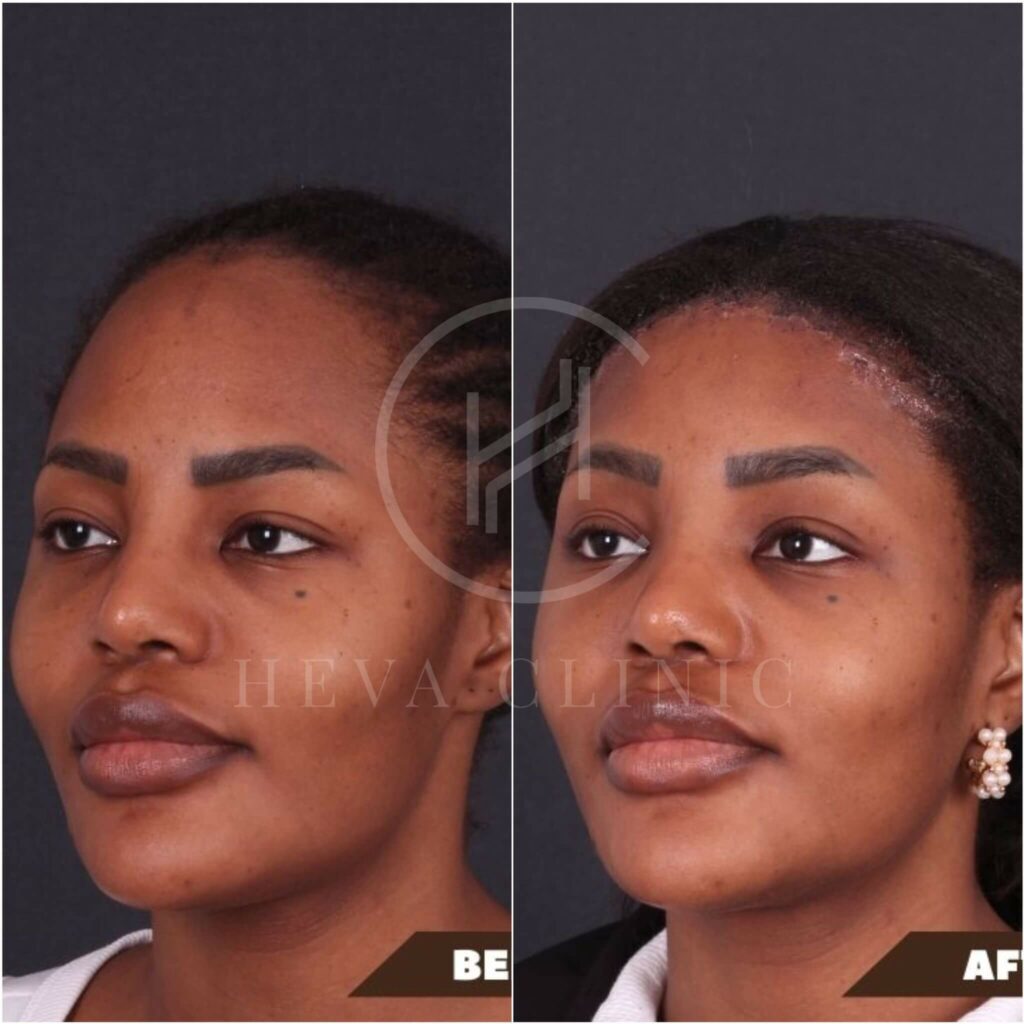The image is a split-screen, side-by-side comparison of before and after photographs of the same dark-skinned woman, set against a dark gray background. The left photograph, labeled "BE" in the bottom right corner, shows her in profile with neatly pulled-back dark hair, dark eyes, and full lips. She is wearing a white shirt, and her face is largely unadorned with a clear focus on her natural features. The right photograph, labeled "AF" in the bottom right corner, features the same woman with noticeable changes. Her hair, no longer pulled back, cascades down the sides of her face, partially covering her forehead. She wears white earrings and seems to have had her eyebrows trimmed, giving her a more styled appearance. In this shot, she is dressed in a white and black top. The entire image is watermarked with the HEVA Clinic logo, featuring a double H within a circle, emphasizing the clinic's involvement in her transformation.